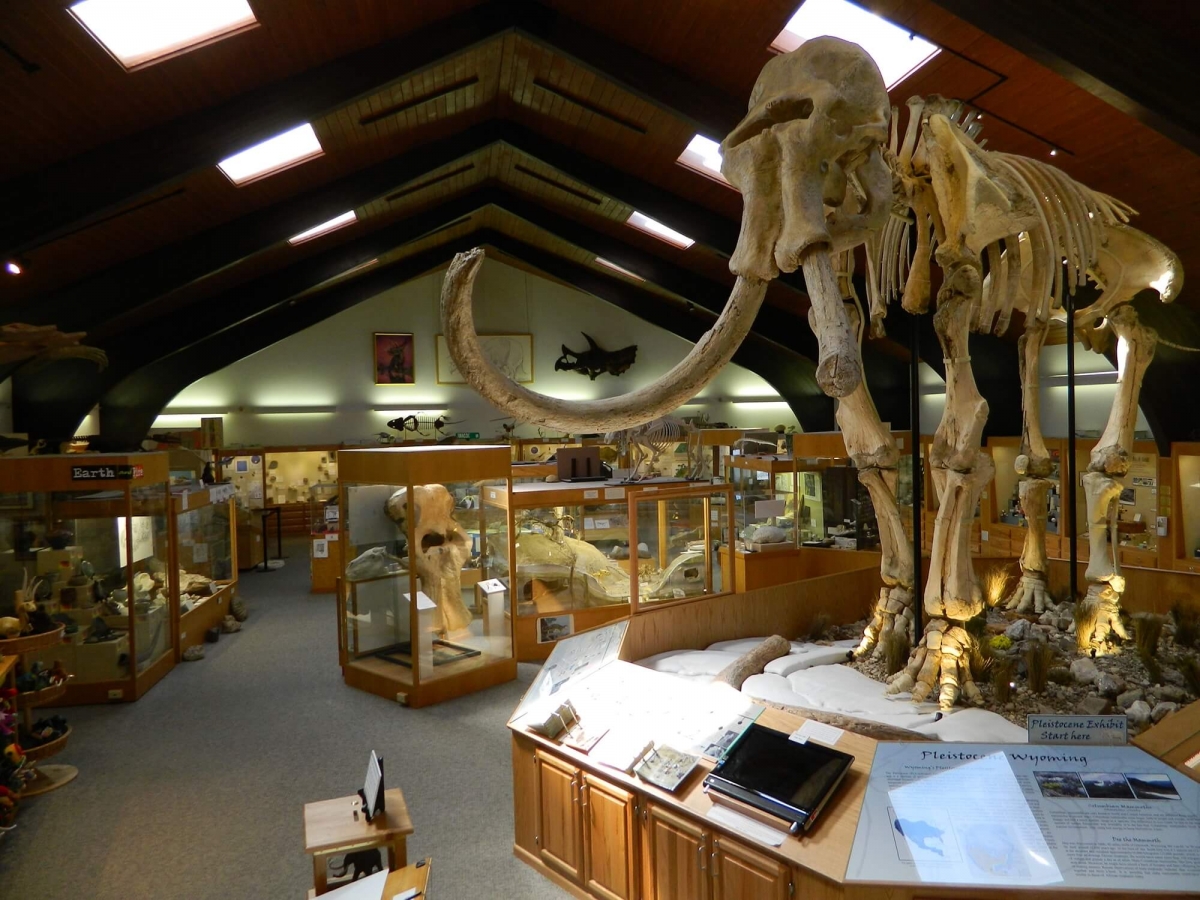In this detailed museum exhibit image, the focal point is an impressive fossilized woolly mammoth, prominently displayed on a stone platform within a wooden exhibit area. The mammoth, with its massive bone structure and single curved tusk, commands attention as the tallest skeleton in the room. Informative placards and a monitor nearby offer educational insights about this prehistoric giant, emphasizing its significance. Surrounding the mammoth, various other fossils and skeletons— including heads of a triceratops, a fish skeleton, and a dog or coyote skeleton—are meticulously arranged in glass cases with wooden frames. A label indicating that the mammoth is from Wyoming ties this exhibit to its geographical origins, enhancing the display's educational value about Earth's ancient creatures.